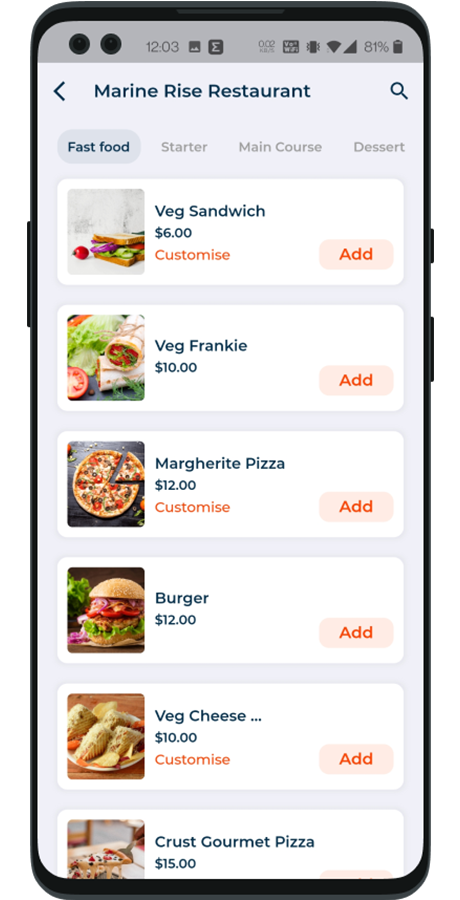A detailed mock-up image showcases a smartphone displaying the menu for Marine Rise Restaurant. The screen captures a wealth of information: starting from the top, the phone's status bar on a light gray background, including a readable time of 12:03 on the left, and essential icons on the right such as an 81% battery level alongside a nearly full battery icon.

The restaurant menu, titled "Marine Rise Restaurant" in dark blue text, dominates the screen. On the left of this heading, there's an arrow-shaped back button, resembling a carrot, also in dark blue and facing left. Adjacent to the restaurant name on the right, a dark blue search icon, illustrated as a magnifying glass, is visible.

Beneath the restaurant title, different menu categories are presented, with "Fast Food" selected. This category is highlighted by a rectangular button with curved edges, featuring dark blue text. Other categories like "Starter," "Main Course," and "Dessert" appear in light gray text, indicating they're not selected.

Under the "Fast Food" heading, various menu options are arranged neatly. Each item is displayed within a white rectangular background, accompanied by food icons or photographs on the left. The menu items include a variety of vegetarian dishes, but a burger image is noticeable approximately halfway down the list. The overall layout provides a clear, organized view of the restaurant’s offerings, enhancing user interaction on the smartphone interface.